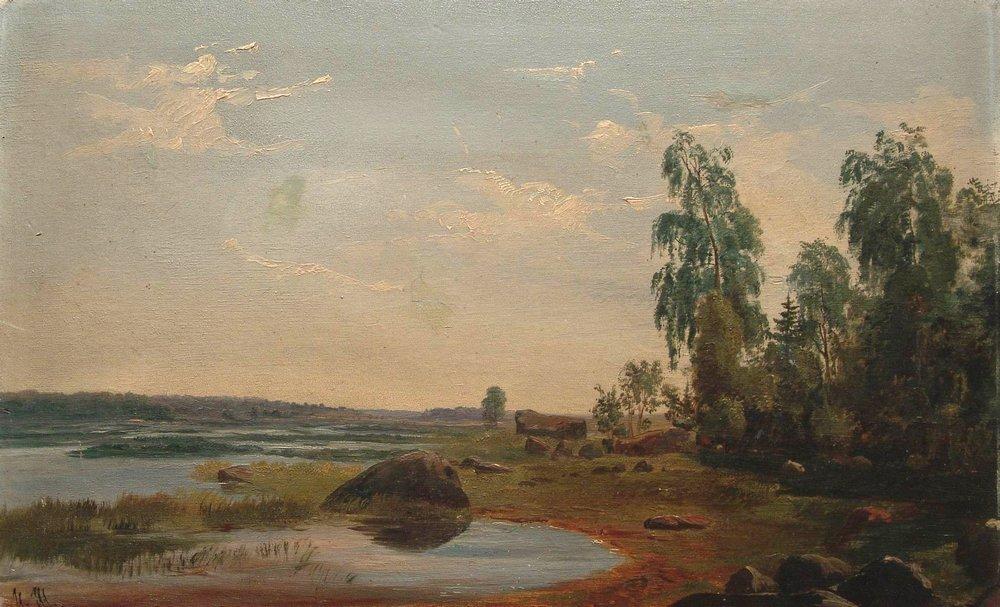This painting, likely created with acrylic or oils, presents a serene yet somewhat unimpressive landscape rendered with meticulous detail. In the bottom center of the composition lies a small, round body of water, bordered by a prominent rock. The water appears to trickle in from the left side, mingling with marshy grass and additional rocks. The landscape transitions into flatland toward the left and includes some brown patches of land, dappled with gray undertones. 

To the right, a cluster of tall and small trees, along with bushes, droop slightly, their foliage displaying a mix of greens and yellows with darker shades at the base. The sky above is a subdued blue adorned with soft white clouds, with some areas appearing as if raw paint was deftly applied without heavy blending, imparting a smoky, gray-beige ambiance to the scene. The grass in the foreground hints at an autumnal shift, retaining patches of green amidst a spectrum of grays. Despite the overall unremarkable nature of the terrain—a juxtaposition of water, rocks, and vegetation—the artist's impressive technique elevates this tranquil landscape, capturing both the simplicity and complexity of nature.